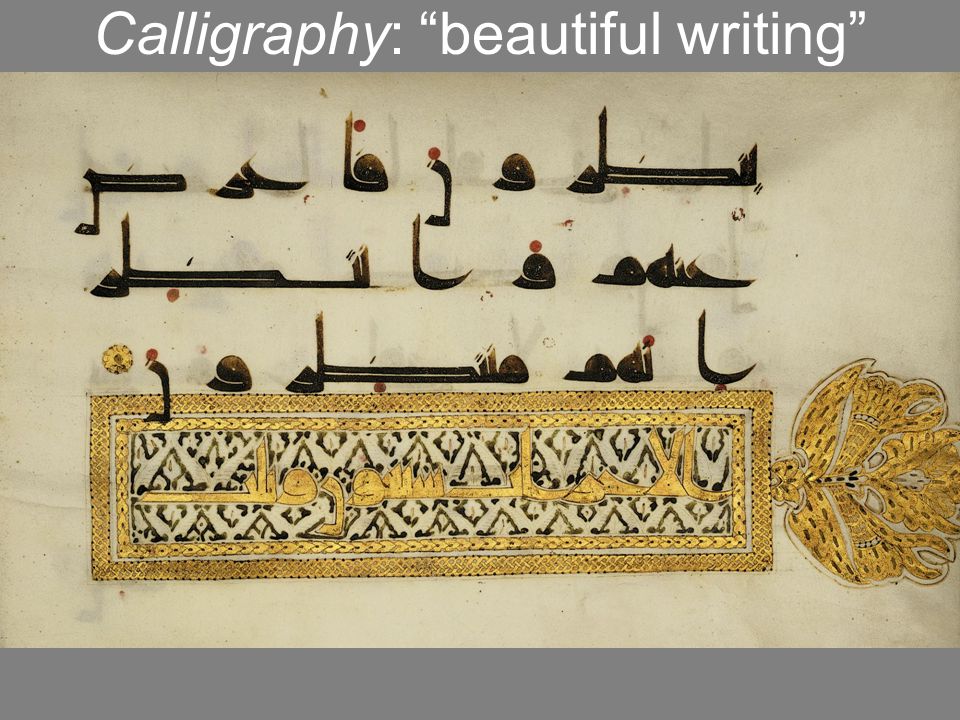The image, titled "Calligraphy: Beautiful Writing," features an elegantly styled photograph of Arabic text. At the top, a dark grey header spans the width of the image, displaying the title in white calligraphy. Below this header, the main portion of the image showcases meticulously detailed Arabic writing in thick black ink, accented with red dots above select letters or words. The background has an off-white, parchment-like appearance, enhancing the text's classic, timeless feel. Towards the bottom of the image, there is a golden rectangular box adorned with intricate floral designs and patterns, particularly a large floral flourish on the right-hand side rendered in gold and black paint. This golden box also contains more Arabic writing in golden paint, adding a layer of visual richness and complexity. The composition is framed at the bottom by another grey footer, which, like the header, extends across the entire width of the image, providing a balanced and harmonious structure.